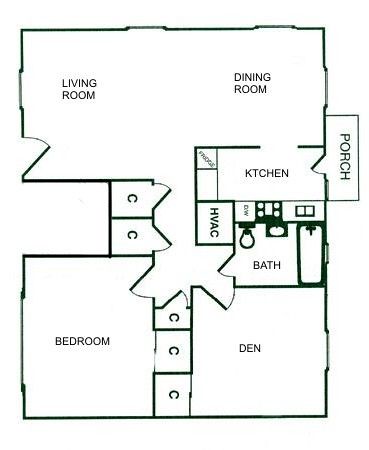This image depicts a meticulously machine-made architectural layout of a square-shaped house or apartment. The detailed floor plan is designed with careful consideration for each room's placement and function. 

Starting from the top left, the spacious living room, which is also square-shaped, features a door that opens directly from the outside. Adjacent to it on the top right sits the dining room, somewhat smaller in size but retaining a similar square configuration, and it includes two windows that allow natural light to flood the space. 

Connecting the dining room to the kitchen is a strategically placed door located directly below the dining area. The kitchen is designed as a rectangle and to its right is a porch, accessible through a door situated within the kitchen. 

Below the kitchen lies the well-equipped bathroom, complete with a bathtub, toilet, and sink. To the left of the bathroom, the HVAC (heating, ventilation, and air conditioning) unit is centrally located for optimal efficiency.

A central hallway runs vertically down the middle of the square-shaped layout. At the midpoint on the left side, two closets with outward-opening doors provide ample storage space. 

In the bottom left corner, the bedroom boasts three closets and a large left-facing window, ensuring plenty of storage and daylight. The bottom right corner houses the den, featuring a medium-sized right-facing window and a door opening into a small hallway. This hallway leads past the HVAC unit to connect the den and the bedroom, ensuring a thoughtful flow and accessibility throughout the home.